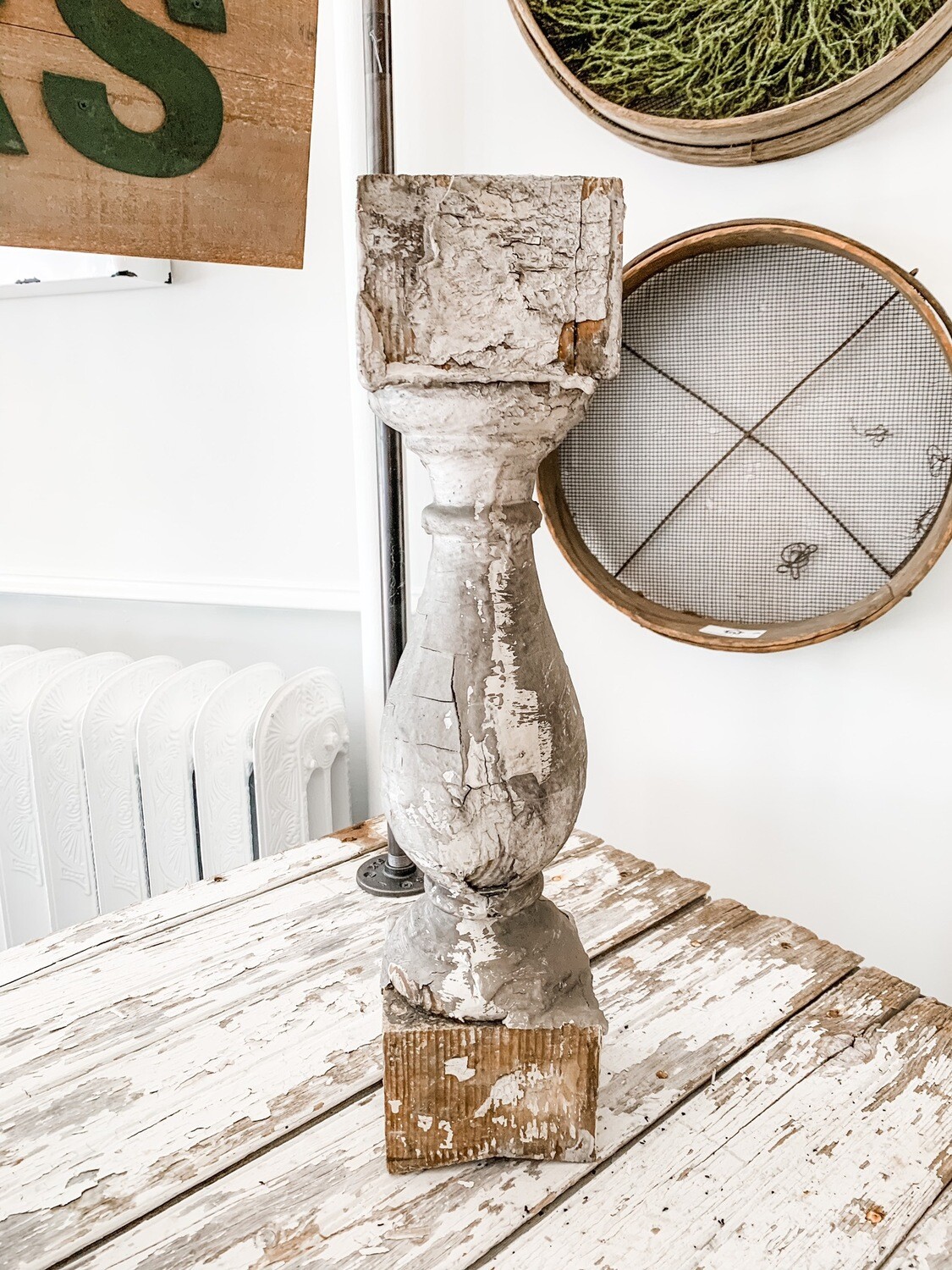The image showcases a rustic, weathered setting within a white room. Central to the image is an old, ashen gray vase or urn, visibly cracked and aged, resting on a wooden block. This block, in turn, sits on a large, heavily worn white-painted table, revealing brown wood beneath due to extensive wear. To the right of this table is the leg of another similarly worn table. The background features a white wall adorned with various items. On one side, a white radiator is visible. Above it hangs a large circular screen with a mosquito net stretched across, forming an X with thin black lines. There are also extra ropes or strings attached to the net's bottom and right quadrants. Above this screen is another circle with a lighter brown rim, containing green, stem-like grass or roots. In the top left corner, part of a wooden sign is visible, showcasing a black letter "S."